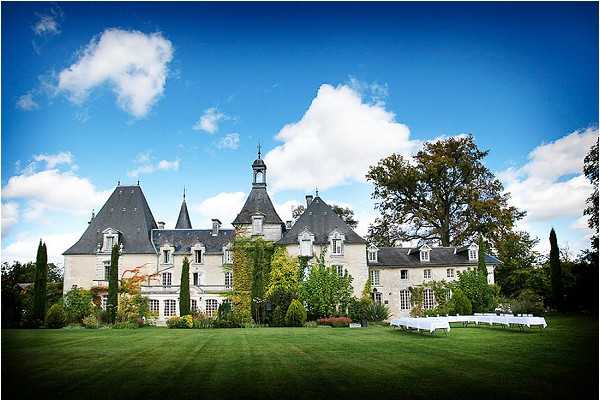The image depicts a large, grandiose white house, perhaps a mansion, characterized by its intricate architecture and steep, varying gray roofs. The house is composed of five connected sections, each with different roof heights, the tallest featuring a clock tower. Multiple embellished window frames adorn the façade, and several chimneys are visible. This stately home is set against a vivid blue sky with ample white clouds hovering above, occupying about half the sky. 

In the background, lush, green trees add to the natural scenery, one standing approximately 50 feet tall with a dense canopy of leaves. The meticulously maintained green lawn in the foreground is complemented by neatly trimmed horizontal shrubs and taller, vertical shrubs about 10 to 15 feet in height. Additional details include an outdoor table setup forming a U shape, adorned with white tablecloths, indicating a possible celebration or event, potentially for a real estate showcase or a wedding venue advertisement.